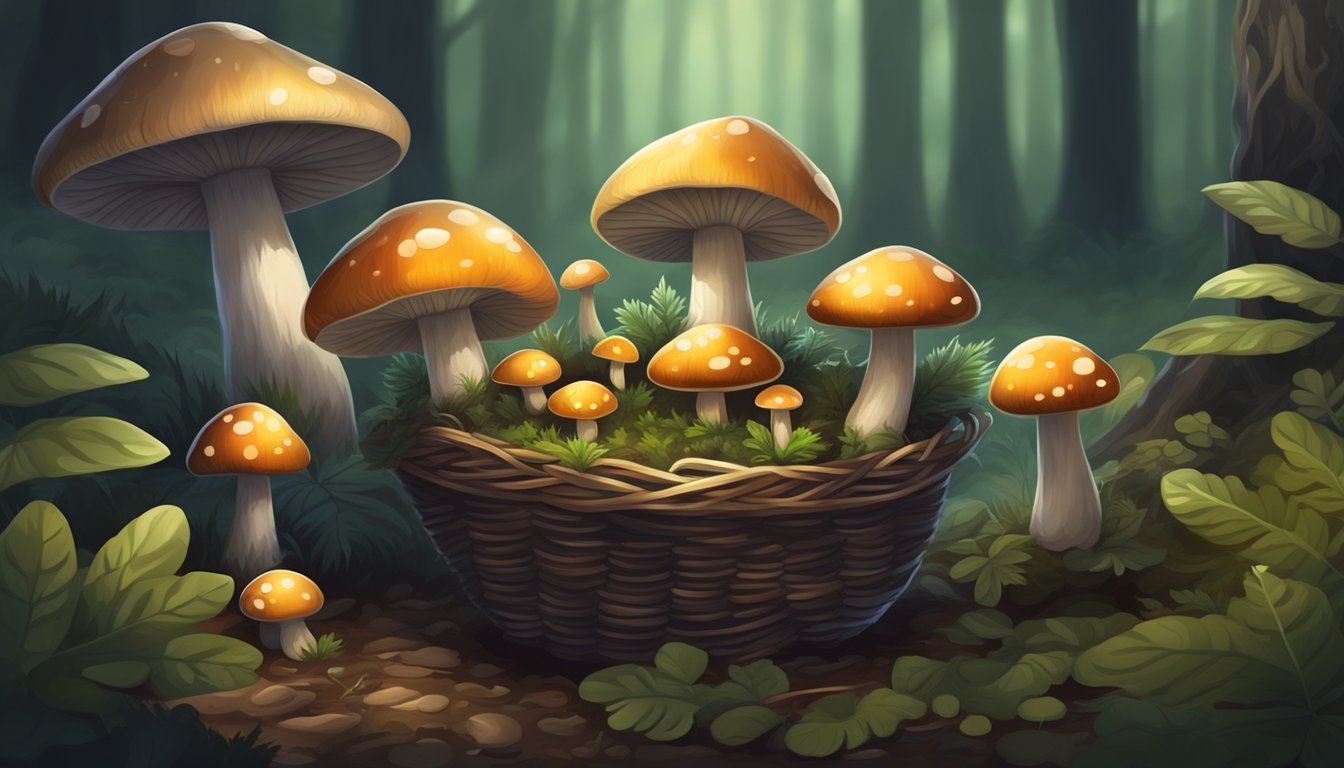This digital artwork features a vibrant, cel-shaded cartoon style drawing of a tan wicker basket filled with lush greenery and mushrooms. Inside the basket, tufts of green grass intermingle with an array of mushrooms – three larger mushrooms and four to five smaller ones. Each mushroom has a white stalk and a cap that transitions from bright yellow to a rich orange hue, adorned with white spots. Surrounding the basket is a background filled with various green leaves. Brown tree trunks and patches of earthy brown dirt frame the scene. Additionally, four mushrooms identical in style to those within the basket are scattered around the outside, completing the whimsical composition.